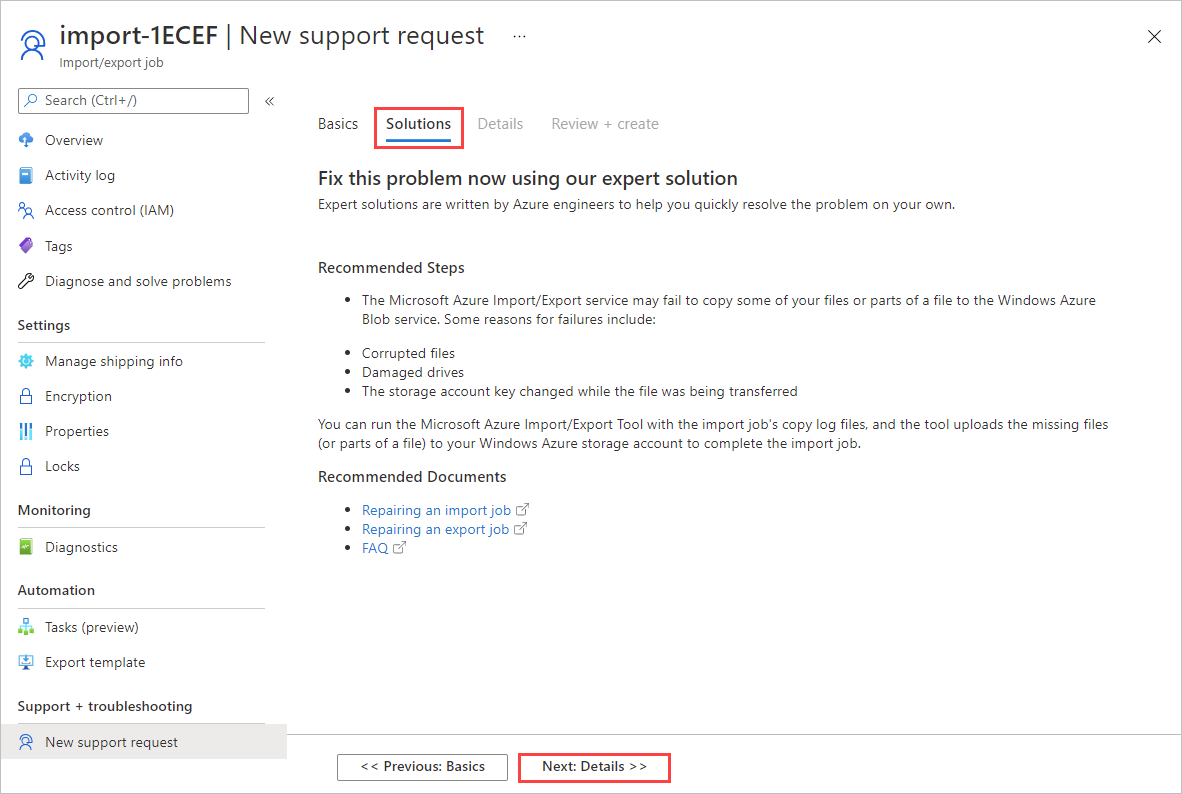In this image set against a white background, the upper left corner contains black text that reads "import 1ecef" with a small grey line running vertically below it. Adjacent to this, there's the text "new support request." Below this section is a search box with the placeholder text, "search," and the shortcut instruction, "control plus forward slash."

To the right of the search box, there's a horizontal navigation menu listing five tabs from left to right: "Basics," "Solutions" (highlighted with a red square around it), "Details," "Review," and "Create." 

Underneath the navigation menu, in bold black print, the text declares, "Fix this problem now using our expert solution." Below this message, in smaller text, it reads, "Expert solutions are written by Azure engineers to help you quickly resolve the problem on your own."

Further down, a bulleted list titled "Recommended Steps" suggests that "The Microsoft Azure Import Export Service may fail to copy some of your files or parts of a file to the Windows Azure Blob Service." The possible reasons for failures mentioned include corrupted files, damaged drives, and changes to the storage account key while the file was being transferred.